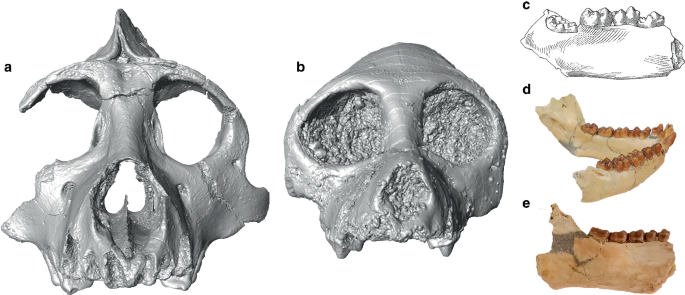This image presents a collection of skull and mandible artifacts, likely replicas, labeled A through E. Artifact A is a fragmented skull, showcasing a largely intact eye socket on the left and a damaged one on the right, alongside partial nasal and dental structures. In contrast, Artifact B features a more complete yet plainer skull with fully filled-in eye and nasal cavities, lacking the intricate damage seen in A. Artifact C is a black-and-white illustration, probably a pen or pencil sketch, displaying a detailed view of teeth and gum. Artifacts D and E, rendered in a brown tone, depict the upper and lower sets of teeth and gums, highlighting various dental structures. These pieces appear to be carefully crafted, giving the impression of a meticulous study likely aimed at educational or archaeological insights.